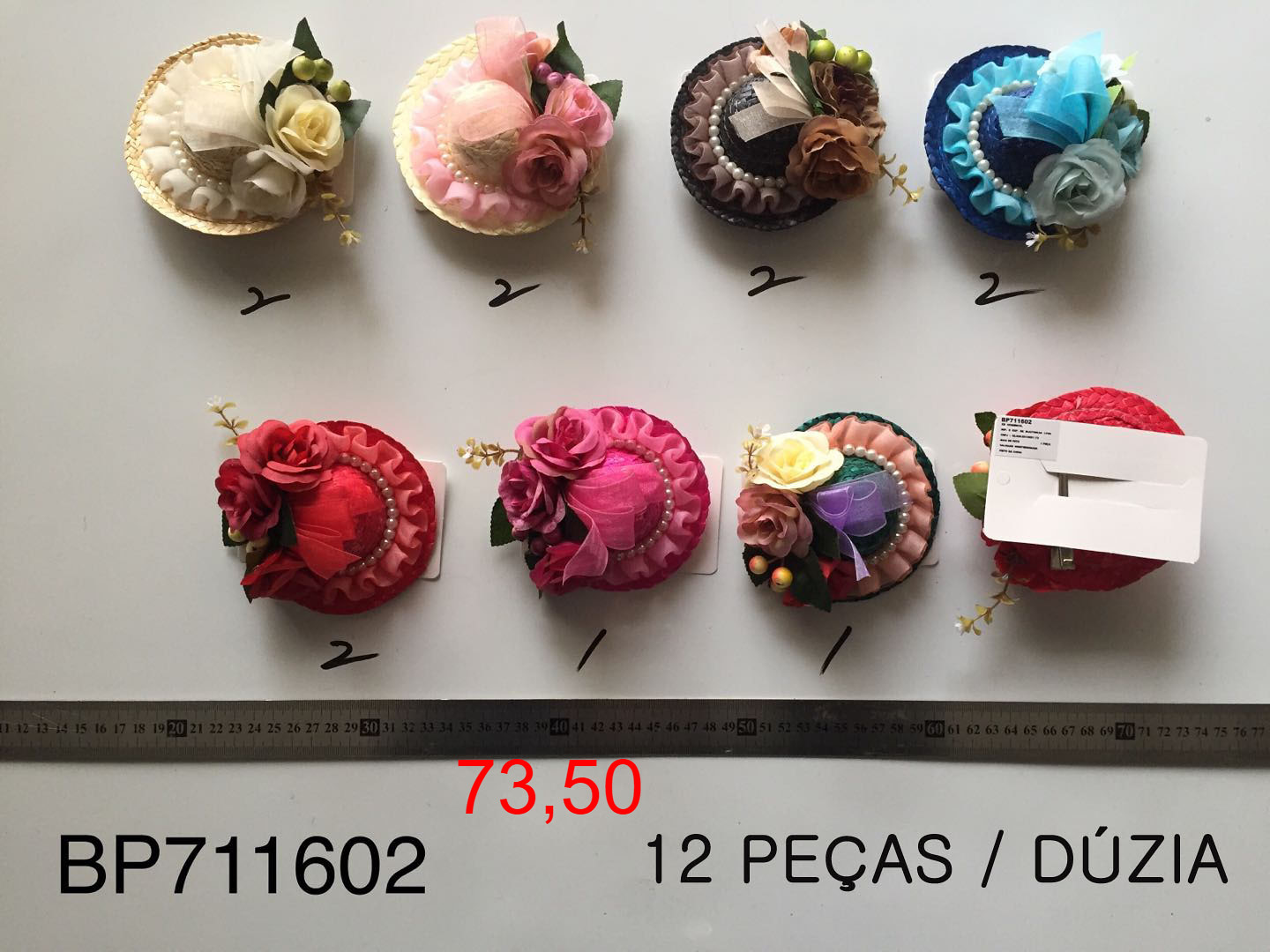This is a professional product photo intended for an online listing. The image features eight intricately designed, round pendants. Each pendant has a colorful, ruffled fabric base adorned with beadwork, ribbon pins, and a central flower. From top left to bottom right, the pendants are described in detail: the first is white with a yellow rose; the second is white with a pink rose; the third is black with a brown rose; the fourth is blue with a matching blue rose; the fifth is red with a red rose; the sixth is bright pink with a pink rose; the seventh is a grayish color with a gray rose; and the eighth, partially obscured by a white square paper with black text, appears to be red.

The background of the image is a bluish-white gradient with black text on both sides. On the left, "BP711602" is visible, and on the right, it reads "12 P-E-C-A-S/D-U-Ñ-C-I-A" suggesting a dozen pieces, likely in Spanish. Near the middle of the image, there’s a red-font price of "73,50" and a silver metal measuring tape with black numbers.